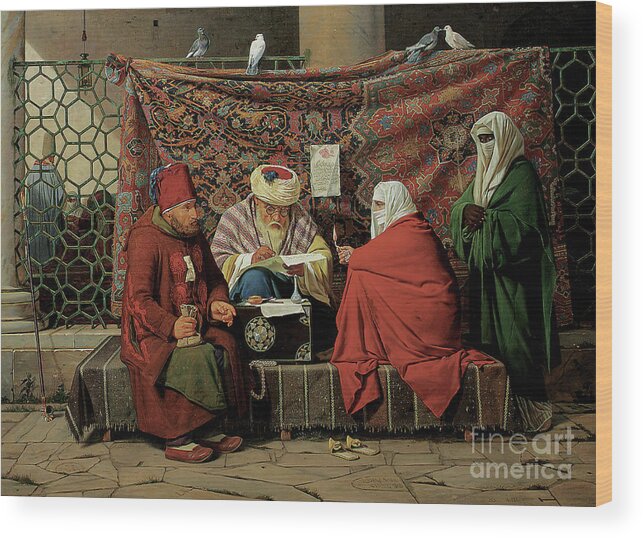This fine art painting, reproduced on an inch-thick wooden slab, features intricate details and vivid imagery captured with meticulous brushstrokes. Positioned along a wrought iron fence adorned with geometric patterns and flanked by stone columns, a large, multicolored Persian rug is draped, adding a rich oriental texture to the scene. Four birds, possibly pigeons or doves, perch on the fence and rug, bringing a touch of life to the composition. 

In the foreground, a merchant, distinguishable by his Santa-like beard, glasses, and a turban, is engrossed in writing on a piece of paper, illuminated by a woman holding a candle. This woman is draped in a long, red cloak-like garment and wears a head wrap that covers her face, embodying the modesty typical of a Muslim community. To her right stands another woman with darker skin, enveloped in a green garment with her head and face similarly covered, revealing only her eyes. 

On the merchant’s left, a man in leather slippers, a tall fez hat, and a red robe sits on a low table holding a small money sack. A mother-of-pearl inlaid chest rests on the table in front of the merchant, enhancing the scene's opulence. The background's concrete-like texture, combined with these rich elements, evokes a sense of historical and cultural depth, signified by the watermark "Fine Art America" in the bottom right corner. 

Every detail, from the attire suggesting an Islamic or Arabic setting to the interplay of light and color, creates a vivid, narrative-driven scene imbued with cultural nuance and artistic elegance.